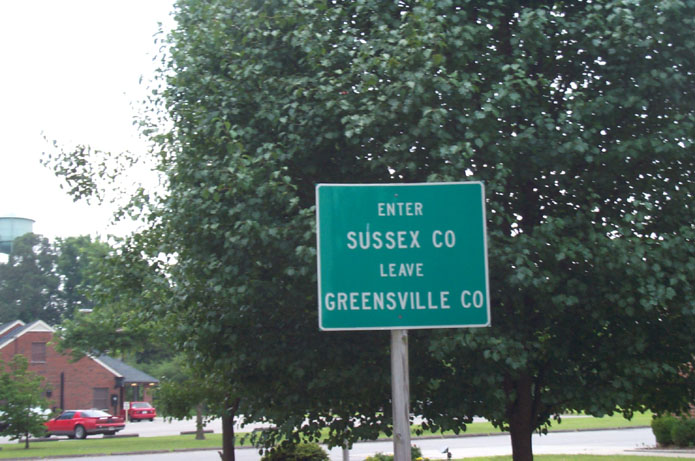The photograph showcases a detailed scene centered around a green street sign mounted on a gray steel pole with white lettering that reads "Enter Sussex County, Leave Greensville County." The sign stands prominently against a backdrop of lush, tall coniferous trees that fill the upper two-thirds of the image. To the left of the sign, a one-story brick building with a dark roof, likely a bank, features a right-handed drive-thru and is accompanied by a parking lot. In front of the building, two red cars are visible — one in the drive-thru and another parked near the entrance, partially obscured by a tree. On the far left, a black SUV is also parked behind the tree. In the further background, behind another set of trees, the top of a light blue water tower can be seen. The bottom part of the photograph includes a portion of the road and some hedges lining its side. The entire scene is bathed in the richness of full foliage, creating a vivid and bustling yet tranquil atmosphere.